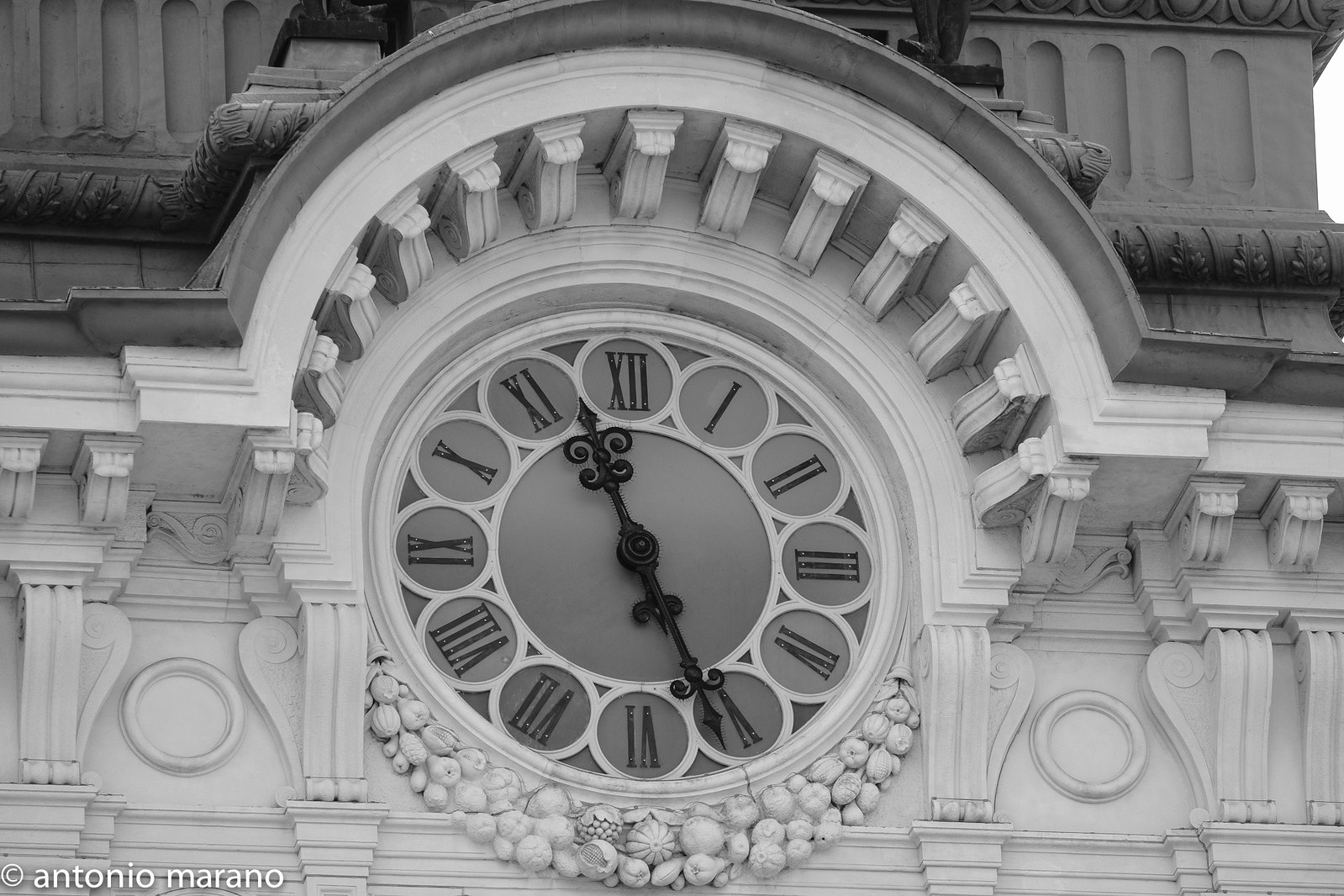This black and white photograph features an ornate clock tower on a building, with intricate details captured in stunning clarity. The building itself is constructed from a white alabaster material, transitioning to dark gray at its upper levels, indicative of concrete. The clock is nestled beneath an arch in the upper part of the structure, which is adorned with thirteen elaborately carved scrolls on its underside. 

The clock has a gray face encircled by large white circles marking each Roman numeral, which are rendered in black. The clock's hands, also black, are exceptionally decorative, resembling wrought iron with intricate scrollwork. Beneath the clock, carved details resembling fruits, vegetables, or seashells add to the elaborate design. The photograph bears the inscription "Antonio Marano" in white letters at the bottom-left corner, adding an artistic touch to this beautiful representation of a historical architectural piece. 

In the background, the building extends upward, with dark gray leaves and ornate decorations carved into its structure, enhancing the clock tower's majestic and timeless appearance. The time shown on the clock is just about a minute to five.